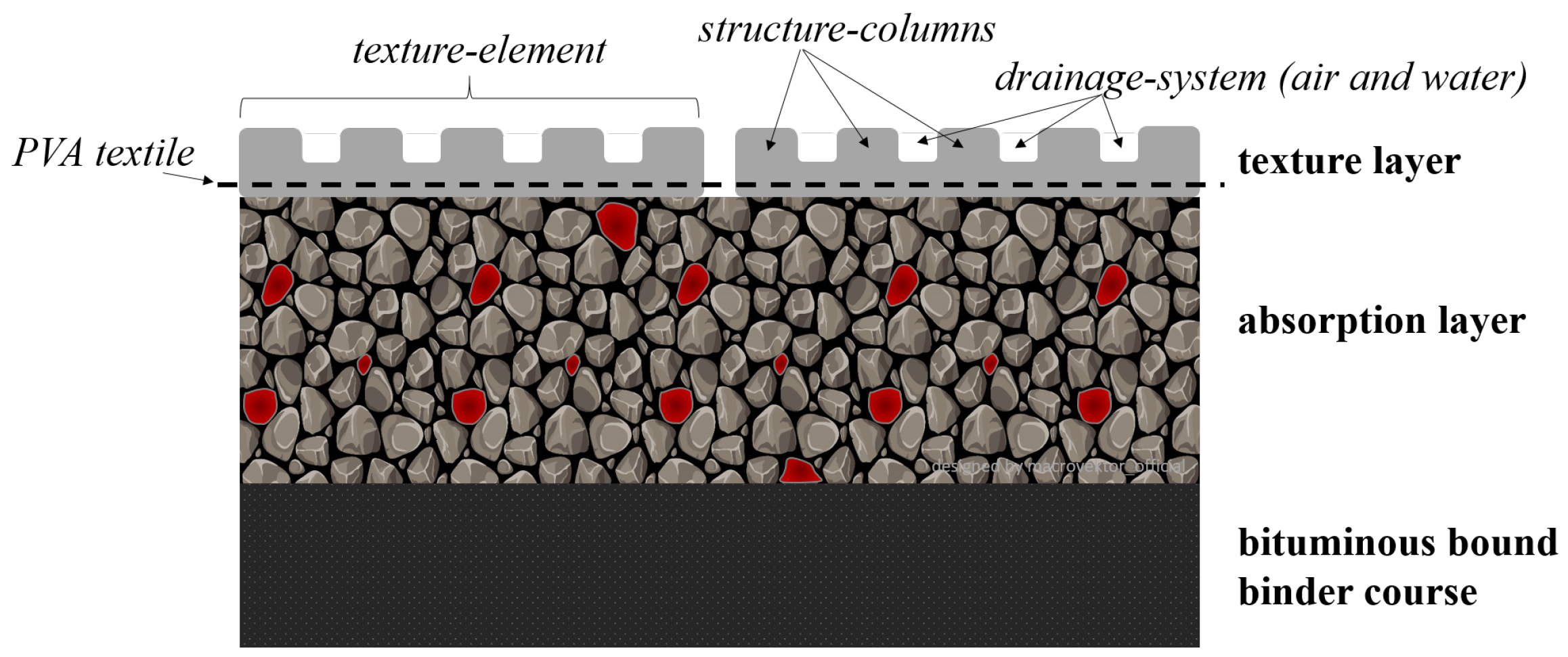This is a comprehensive graphic illustration typically found in educational resources, such as textbooks or online courses, explaining the components and structure of insulation systems. The image is a detailed cross-section of a rectangular insulation layer, featuring multiple labeled segments, each pointing to distinct layers and elements within the rectangle.

At the bottom of the rectangle, you will find a charcoal gray section labeled "Bituminous Bound Binder Course." Above this layer, there's an "Absorption Layer," depicted as tightly packed gravel with interspersed red gravel pieces. Moving upwards, you encounter the "Texture Layer," characterized by a light gray color with ridges resembling square sine waves.

On the far left side of the graphic, an arrow points to a dotted line traversing the top of the rectangle, labeled "PVA Textile." Across the top of the image, another label reads "Texture Element," with a bracket-like arrow encompassing the square bumps and gaps in between them. Within the mid-section of the rectangle, the term "Structure Columns" directs attention to the individual square bumps, while the label "Drainage System (Air and Water)" specifies the purpose of the gaps between these bumps.

Overall, this intricate diagram effectively delineates the multilayered composition and specific functions of each section in the insulation system.